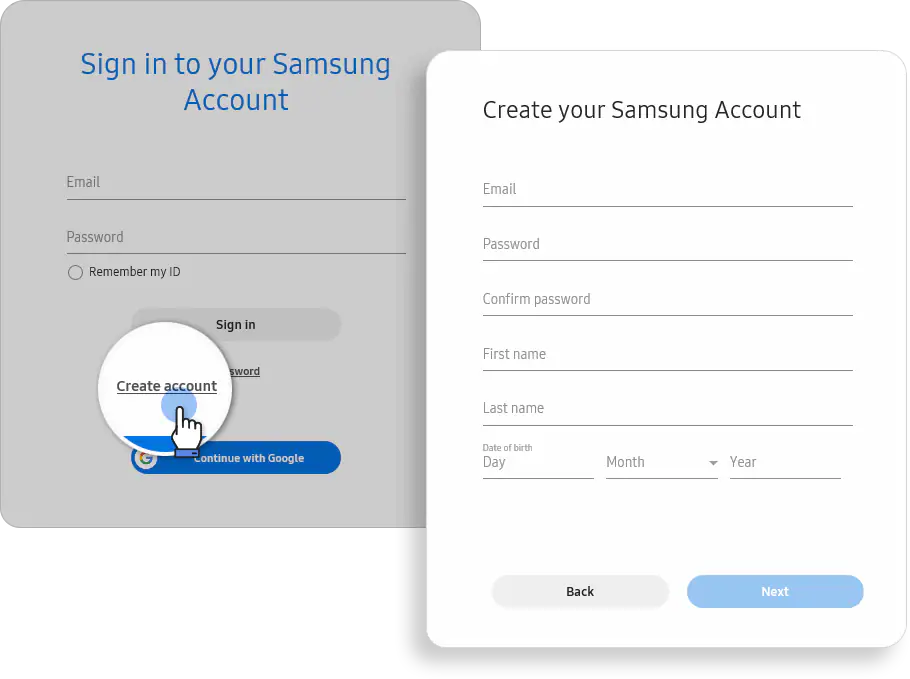The image depicts two overlapping pop-up tabs side-by-side, with the tab on the right slightly overlapping the tab on the left, creating a distinct gray overlay effect on the left tab where they intersect. 

**Left Tab:**
- The left tab features a gray hue due to the overlap.
- It features a header in bold blue lettering at the top center that reads "Sign into your Samsung account."
- Below the header:
  - The word "Email" is in black lettering, followed by a black underline.
  - The word "Password" is in black lettering, followed by a black underline.
  - To the right of these fields is an outlined black circle with the text "Remember my ID" in black.
- Below these fields, there is a gray button with the text "Sign in" in black lettering.
- Further down, there is an underlined word in black that appears truncated due to the overlap of the tabs. There is a white circle with a black "Create account" text over this word, suggesting an interactive element.

**Right Tab:**
- The right tab prominently displays a white background.
- At the top, in large black lettering, it says "Create your Samsung account."
- Below this heading:
  - In smaller black lettering, the label "Email" with an underline extending the width of the tab.
  - Similarly formatted labels for "Password," "Confirm Password," "First Name," and "Last Name," each with respective lines underneath.
- The bottom corner features: 
  - A gray button on the left side with "Back" in black lettering.
  - A blue button to the right with the text "Next" in white lettering.

Together, these overlapping tabs create a clear visual distinction between signing into an existing account and creating a new Samsung account with distinct, easy-to-follow input fields and interactive buttons for user engagement.